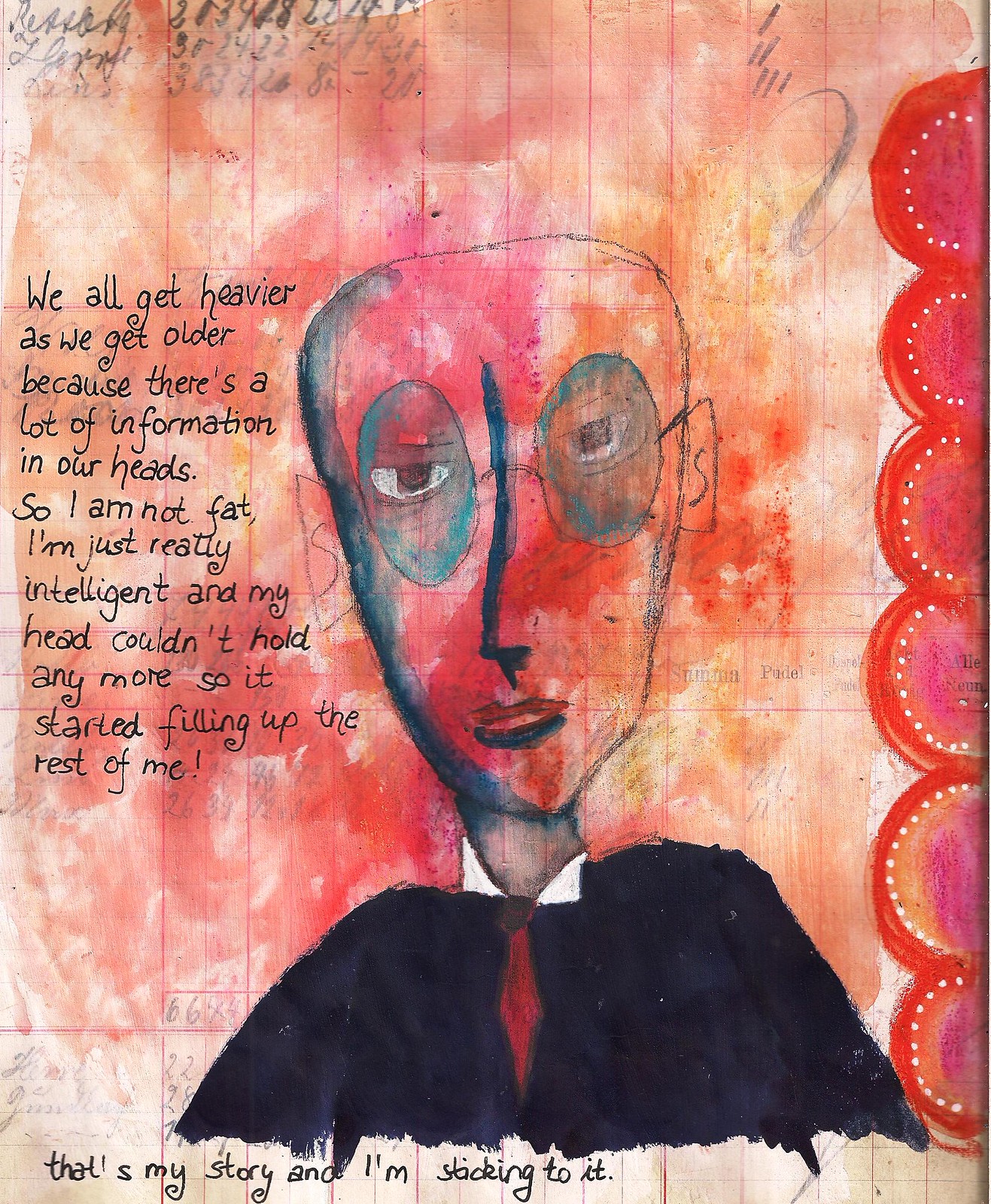This captivating image depicts an abstract, almost cartoon-like painting of a person situated at the center of the composition. The figure, which appears to be a bald-headed person with a suit and a short red tie, could be interpreted as either a man or a woman due to its stylized features. Wearing glasses, the person is portrayed with striking shades of green, pink, red, and orange, adding to the vibrant, watercolor-esque quality of the artwork. 

On the left side of the image, there is an intriguing text that reads, "We all get heavier as we get older because there's a lot of information in our heads. So I'm not fat, I'm just really intelligent, and my head couldn't hold any more, so it started filling up the rest of me. That's my story, and I'm sticking to it." The text is positioned with a pencil-like handwritten style, complementing the artistic feel of the piece.

Adding to the visual interest, the right-hand side of the painting features a decorative element: a series of red circles with white dots encircling them, running vertically from top to bottom. This graphic pattern balances the overall composition, making it a visually stimulating and thoughtful piece of art.